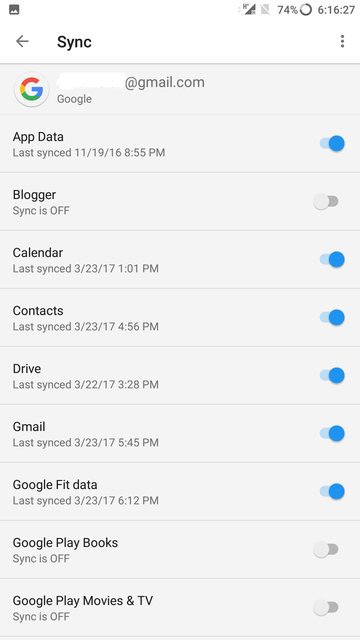The image is a screenshot taken from a smartphone, featuring a synchronization settings screen for a Google account. 

At the top of the screenshot, there's a white border, with the battery percentage displayed at 74%. The time is shown as 6:16:27. Towards the left, there's a left-pointing arrow next to a "Sync" heading. 

The primary part of the screen has a gray background. In the upper left corner, the Google "G" logo is visible, adjacent to a text field meant for entering an email, displaying a placeholder as "blank@gmail.com". 

Below this, a vertical list of synchronization options appears, each with a toggle switch and relevant information about the last sync time. 

- **App Data**: Last synced on 11-19-16 at 8:55 PM, toggle switch is on (highlighted in blue).
- **Blogger**: Sync is off.
- **Calendar**: Last synced on 3-23-17 at 1:01 PM, toggle switch is on (highlighted in blue).
- **Contacts**: Last synced on 3-23-17 at 4:56 PM, toggle switch is on (highlighted in blue).
- **Drive**: Last synced on 3-22-17 at 3:28 PM, toggle switch is on (highlighted in blue).
- **Gmail**: Last synced on 3-23-17 at 5:45 PM, toggle switch is on (highlighted in blue).
- **Google Fit Data**: Last synced on 3-23-17 at 6:12 PM, toggle switch is on (highlighted in blue).
- **Google Play Books**: Sync is off.
- **Google Play Movies & TV**: Sync is off.